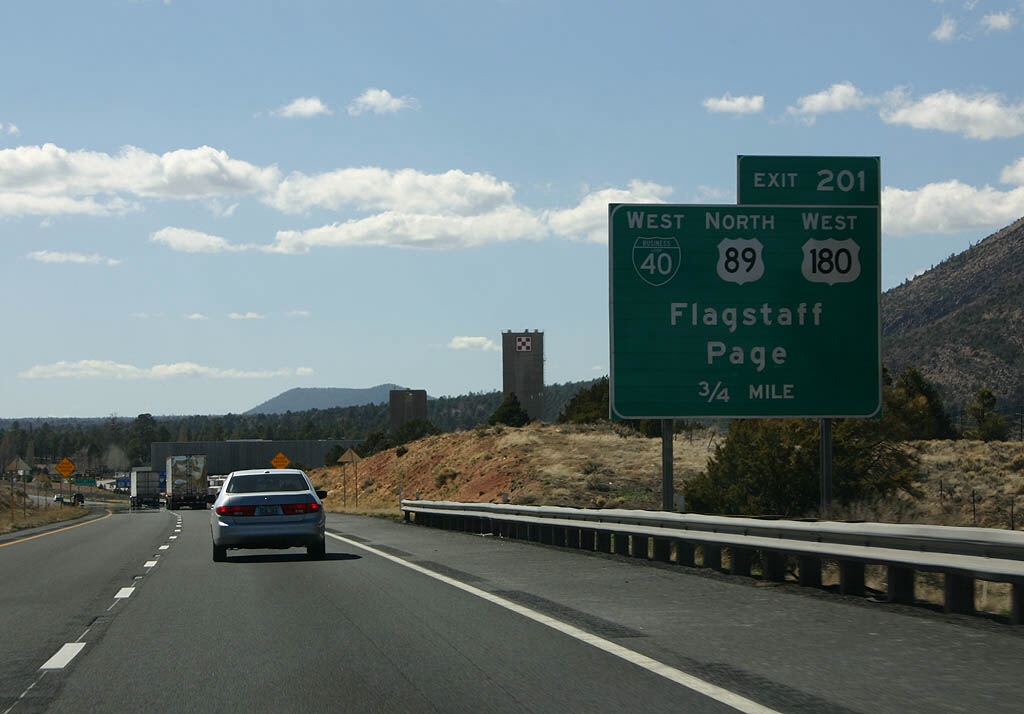The photograph captures a detailed and vibrant highway scene, presented in landscape orientation. The central focus is a stretch of the interstate, with various vehicles, including silver sedans and large trucks, traveling on the right side. Prominently visible on the right side of the image is a green road sign providing directions: "Exit 201," and the routes "West Interstate 40," "North 89," and "West 180," leading towards "Flagstaff" and "Page," indicated to be three-quarters of a mile ahead. The road surface is a stark black asphalt, contrasting with the vivid greenery of hillsides and distant mountains that frame the road. The sky above is clear, showcasing a brilliant blue hue with scattered white clouds, adding to the scenic backdrop. This composition reflects the realism of a bustling freeway captured in a freeze-frame, with the perspective likely from within a moving vehicle, observing other cars and trucks ahead, and the expansive natural horizon beyond a circular barrier wall.